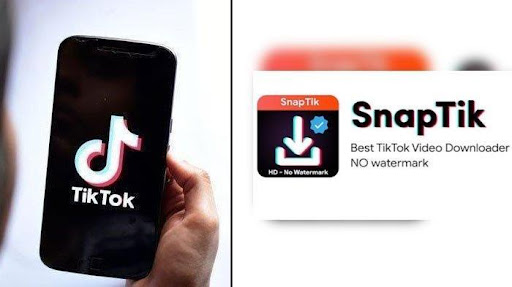The image is divided into two sections by a thin vertical black line. On the left side, there's a photograph of a black smartphone displaying the TikTok logo prominently in the middle of the screen. The logo consists of the word "TikTok" in white, traditional font, accompanied by the iconic backward "J" shaped symbol in a curved design. The phone is held in a person's right hand, with their thumb visible against the side, and the device rests on their palm. The background behind the phone is plain and white, creating a clean, uncluttered look.

On the right side of the split image, the background is slightly blurred but primarily white with hints of red and black tones. In sharp contrast to this backdrop, a popup window is displayed with a header in a red border that reads "SnapTik" beside a blue verified checkmark. Beneath the header, in bold black text, the message "Best TikTok video downloader with no watermark" is visible. There is also an indication that the downloader supports HD videos without watermarks, making it clear that SnapTik specializes in providing high-quality, watermark-free video downloads from TikTok.